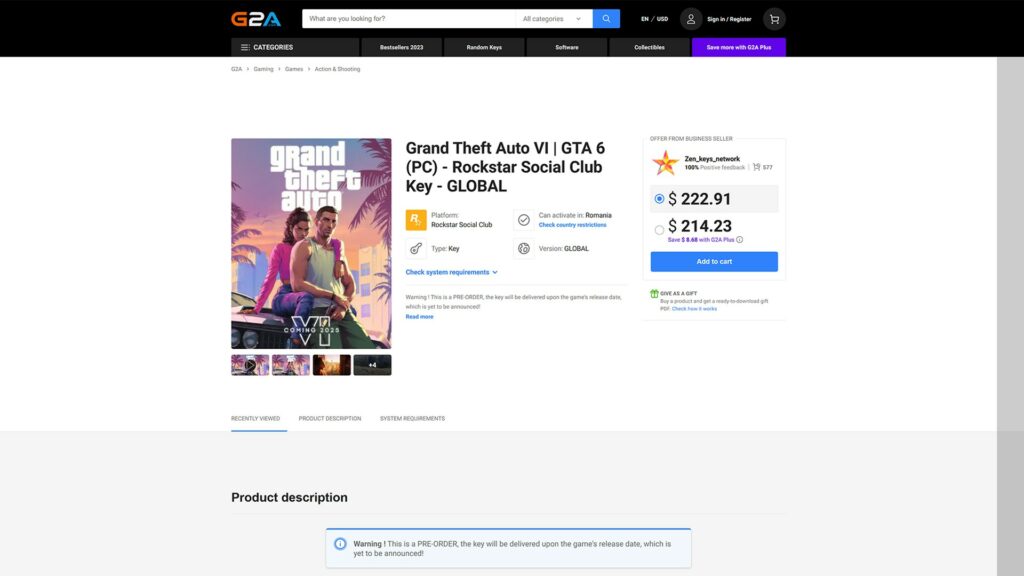The image is a detailed screenshot of a website's header and a selected category. At the top of the screenshot, there is a sleek, black horizontal bar. Centrally positioned within this bar are the stylized letters "G," "2," and "A," each in different colors: red for the "G," white for the "2," and blue for the "A." To the right of these letters is a white search bar containing the text "What are you looking for?" in a light black shade, followed by a dropdown option labeled "All categories" in the same font color, next to a downward-facing "V" symbol. Beside the search bar, a vivid blue box features a white magnifying glass icon.

Further to the right, the header includes a section displaying "EN/USD" in white text and an icon of a person within a circle, which is followed by the options "Sign In" and "Register." Another circle contains a shopping cart icon.

Below this, six different categories are listed horizontally. The sixth category is highlighted in bright blue with white text, indicating it is the selected option. The chosen segment prominently showcases an image of the "Grand Theft Auto" game cover, which is styled to evoke an old Hollywood theme. In this image, a woman is depicted sitting on a car while a man stands in front of her, contributing to the classic cinematic ambiance.